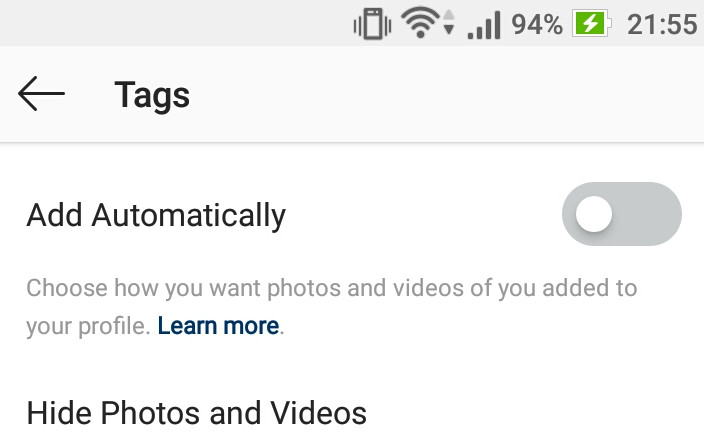This image is a detailed screenshot of a website interface. At the top of the screen, there is a light to medium gray banner displaying several icons. From left to right, these icons include a rectangle with vibrating lines around it, a Wi-Fi icon with up and down arrows (with the down arrow being darker), a cell signal icon, a battery icon indicating 94% charge with a green battery and a lightning bolt symbol, and the time displayed as 21:55.

Below this banner, on the left side of the screen, there is a left-pointing arrow icon followed by the word "Tags" in black print, with a capital 'T'. Beneath this, the background transitions to white. The next feature is an option labeled "Add Automatically" with both 'A’s capitalized. To the right of this option, there is an oval toggle switch which is currently turned off, indicated by a white circle on the left side of the oval.

Further down the screen, there is a description that reads, "Choose how you want photos and videos of you added to your profile." This text is followed by a navy blue link with the phrase "Learn More," capital 'L'. Just below this, another option labeled "Hide Photos and Videos" appears, with the words "Hide," "Photos," and "Videos" capitalized.